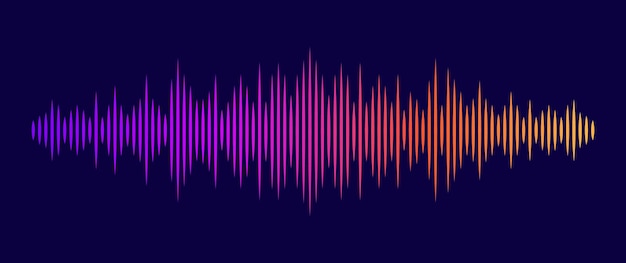This image depicts a vibrant and dynamic audio wave graphic set against a dark navy blue rectangular background. The audio wave, representing an equalizer sound wave pattern, spans horizontally across the center of the image, featuring vertical lines of varying heights. The wave starts narrow and short on both the left and right edges, becoming increasingly taller and more prominent towards the center before tapering off again. The color gradient of the wave transitions beautifully from dark purple on the left, through lighter purples, pinks, and reddish purples, eventually shifting to oranges and ending in a yellowish hue on the right. The tallest, most jagged lines are centrally located, creating a striking focal point in the middle of the graphic. The entire composition captures the essence of an audio recording, visually representing the ebb and flow of sound waves.